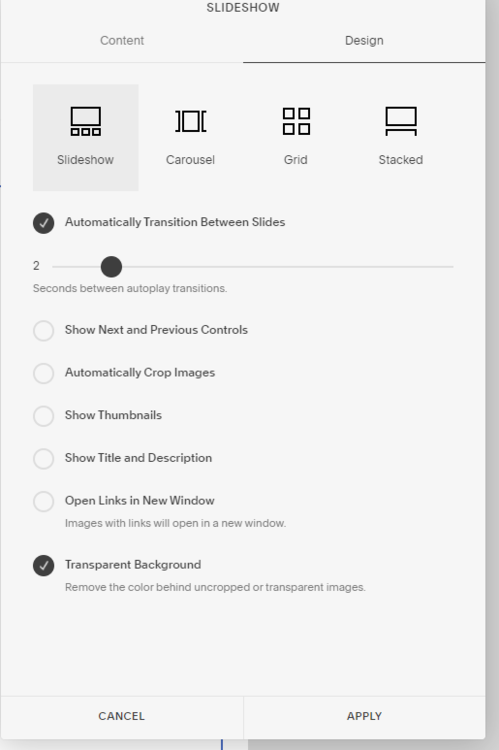The screenshot features a predominantly vertical layout. At the very top, centered against an off-white, light-gray background, the word "Slideshow" is displayed. A darker gray bar extends along the right edge and halfway across the bottom of the screen.

In the top section, there are four distinct icons representing different layout options: slideshow, carousel, grid, and stacked. Directly below these icons, two tabs labeled "Content" and "Design" are visible, with the "Design" tab currently selected, indicated by an underlying line.

The "Slideshow" layout option has a surrounding lighter or darker gray, indicating it is the active choice. Below this, there's a black checkmark accompanied by the text "Automatically transition between slides." Following this, a bar with a black circle on it appears, with the number "2" positioned to the left.

Continuing down, a list of options is presented, each with a circle next to it. The last option, labeled "Transparent background," is selected as indicated by a blackened circle with a check mark. A brief description of this option is provided beneath it.

At the very bottom of the screen, two large buttons occupy half of the width each. The left button reads "Cancel," while the right button is labeled "Apply."